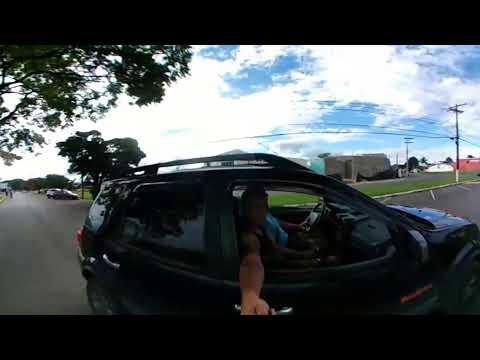This detailed photograph captures a four-door black SUV, possibly a Jeep, equipped with a ski rack on its roof, driving down a road that traverses a mix of residential and business areas. Dominating the frame is a man in a short-sleeved shirt extending his arm out of the window, likely holding a selfie stick to capture a video or picture. The sky overhead is a vivid blue, dotted with patchy white clouds. Around the vehicle, there are visible parking spaces, telephone poles, and several cars on the road. The scene also includes trees both beside and behind the car, with one tree just passed on the left and partial views of buildings and additional trees in the background. The image has a slightly stretched appearance horizontally and is somewhat dark in tone, contributing to a low-quality look where fine details are harder to discern.